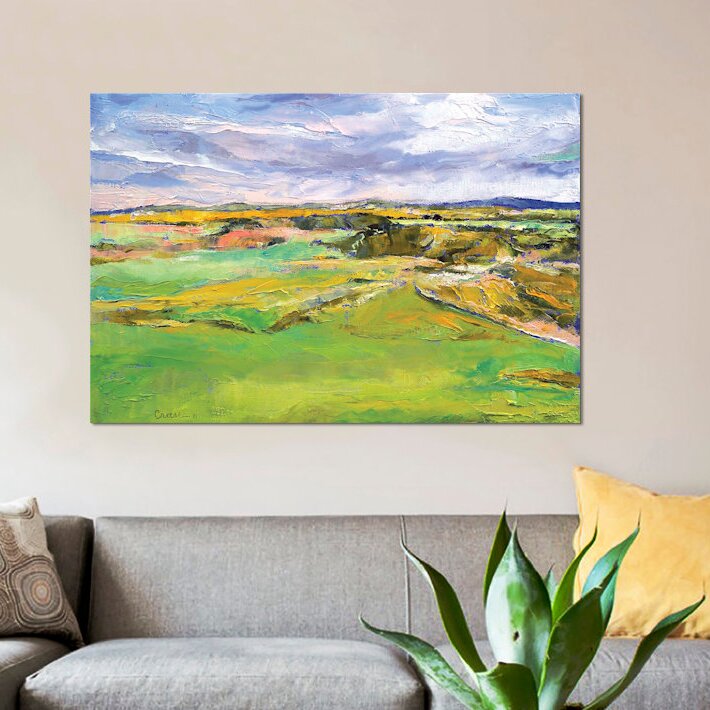The image depicts a modern, minimalist living room with clean, uncluttered design elements. Central to the composition is a gray sofa boasting three cushions, although only parts of the middle and right cushions are fully visible. Adorning the sofa are two distinct throw pillows: one on the right in a vibrant yellow and another on the left, partially visible, featuring a neutral-toned pattern with round, radiating designs. In the foreground, a lush green plant with broad, teardrop-shaped leaves adds a touch of nature to the scene. Hanging on a cream-colored wall above the sofa is a striking landscape painting with an impressionistic style, showcasing a blue sky with clouds, a mountainous terrain with yellowish peaks, and a grassy area in the foreground. The painting highlights natural beauty and complements the serene, modern ambiance of the room.